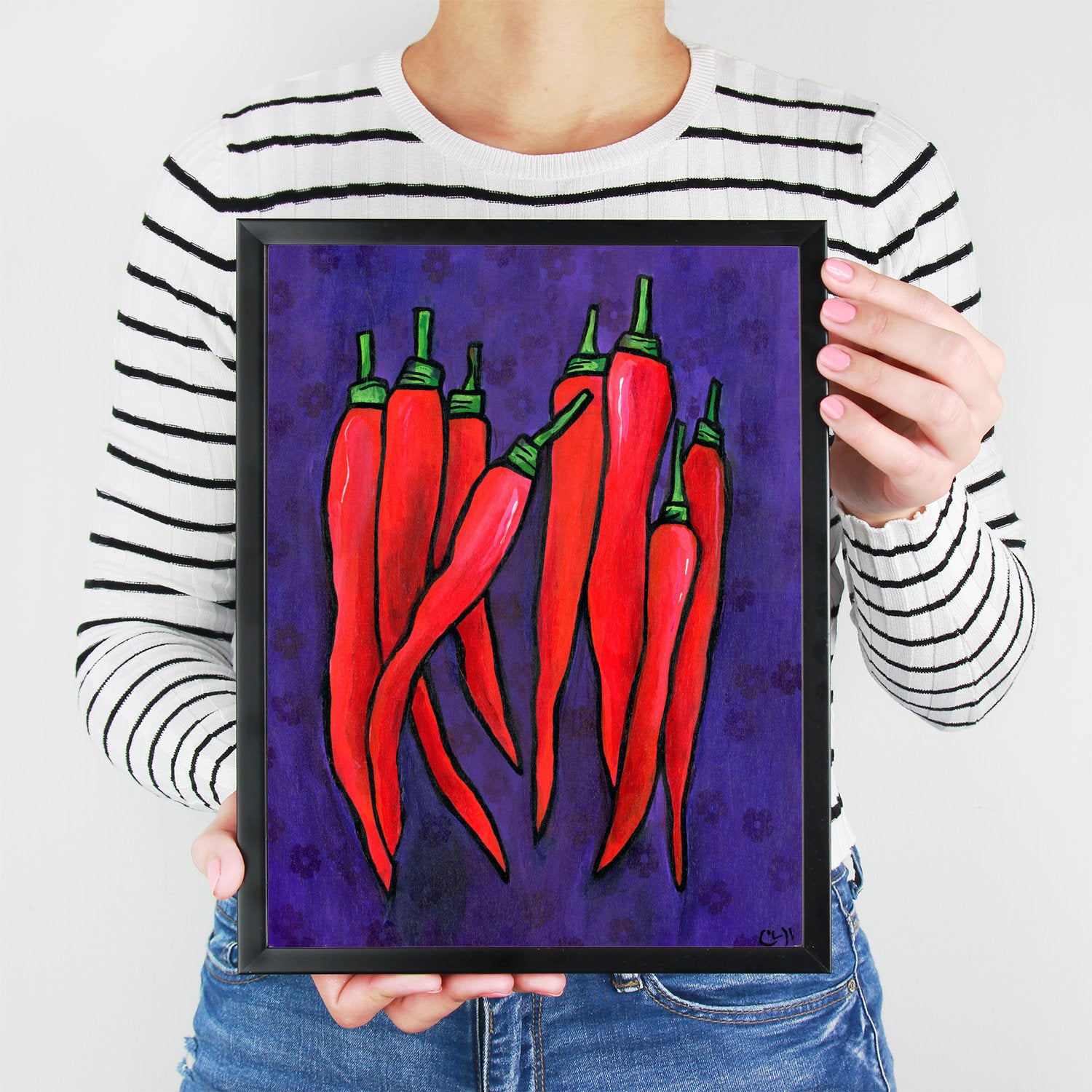In this vibrant full-color photograph, a Caucasian woman holds up a vertically rectangular painting against an off-white background, likely a wall. The image only shows the woman from her neck down to her hips, revealing her white skin, blue jeans, and a long-sleeved white shirt adorned with thin horizontal black stripes. Her pink nail polish adds a pop of color to her extended hands, which grip a black-framed painting.

The painting itself features a deep blue to dark purple background, accented by subtle darker purple or black floral patterns. The primary focus of the painting is a vivid arrangement of eight red chili peppers with green stems. These peppers vary in height and direction: three are clustered together, one leans to the side, another two are grouped, one is noticeably shorter, and one stands slightly taller than the shortest. Despite the intricate details, no artist signature is visible on the painting.